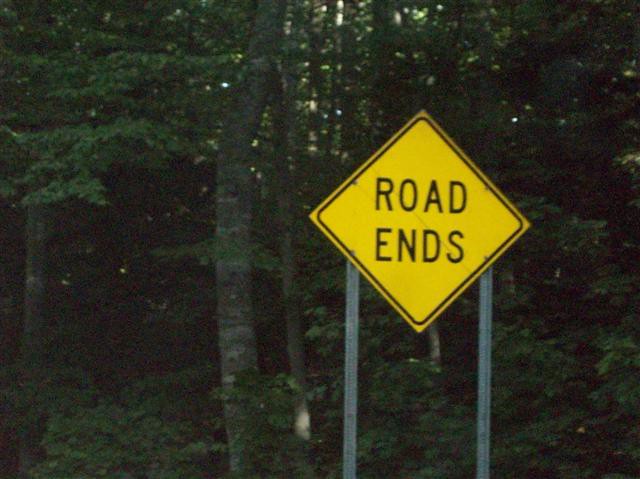In this detailed photograph captured in front of a dense woodland, we see a multitude of green leaves and shrubbery creating a lush, verdant scene. The forest is dense, with gray trees featuring peeling bark that stretches upwards. Sunshine filters through the canopy, illuminating the foreground while the background remains darker, emphasizing the depth of the woods. Prominently displayed at the forest's edge is a bright yellow diamond-shaped road sign bordered in black, with the black lettering "ROAD N" at its center. The sign is mounted on two silver metal poles anchored into the ground, standing in front of a rustic fence. Among the trees, one stands out with a notably crooked trunk, contributing to the natural intricacies of the forest scene.